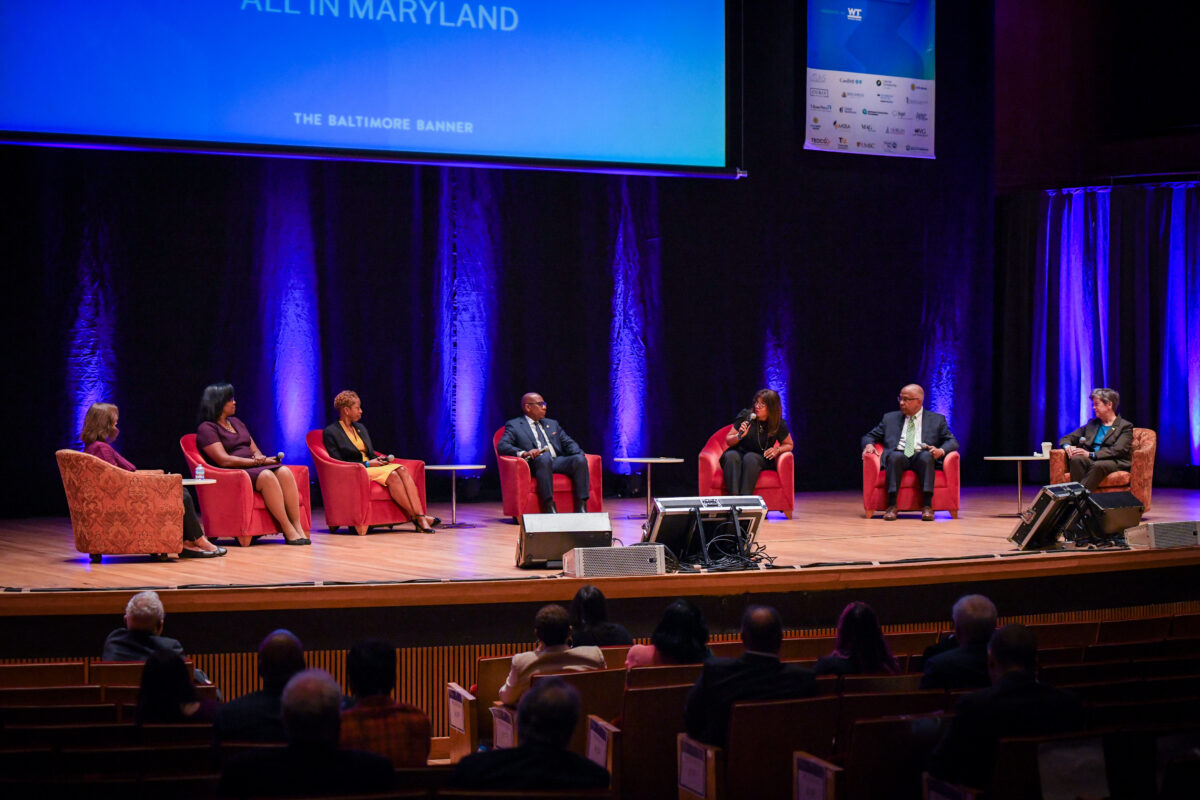On a stage decorated with streaks of bright purple and blue fluorescent lights, seven formally dressed individuals are seated in a semi-circle, engaged in discussion. The backdrop features a partially visible screen displaying "All in Maryland" and "The Baltimore Banner". The participants include three women on the left: one in black pants and a purple shirt, another in a purple dress with black hair, and the third in a yellow dress with a black coat. At the center is a bald black man in a blue suit. To his right, a woman dressed in black holds a microphone, followed by a man in a blue suit with a green tie, and a man on the far right wearing a dark black coat with a blue shirt. Rectangular displays are positioned on the floor in front of them, and small rounded tables are placed between each chair. The audience, sparsely seated and dressed formally, can be seen from behind. This scene takes place during a conference, likely focused on Maryland and potentially political in nature.